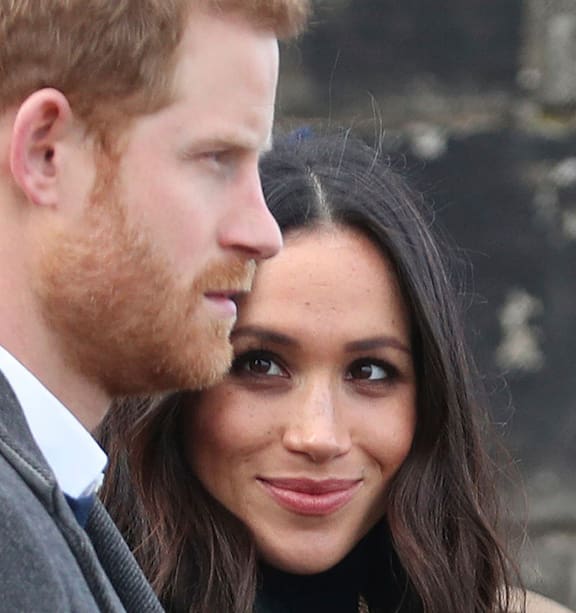The image is a close-up photograph capturing Prince Harry and Meghan Markle. On the left, Prince Harry is shown in profile, facing to the right, with the right side of his face visible. He has a full red beard, short red hair, and a concerned or slightly frowning expression. He’s dressed in a dark gray suit jacket, a white collared shirt, and what appears to be a blue tie. Meghan Markle stands slightly behind him, facing the camera directly. She has long, brunette hair parted at the center, brown eyes, and tanned skin, with minimal makeup—just eyeliner, mascara, and possibly lip gloss. Meghan has a black turtleneck on, creating a dark silhouette under her chin. She is looking up at Prince Harry with a warm, closed-mouth smile, appearing to be very happy and in love with him. The background is out of focus and dark, making it difficult to discern any details.